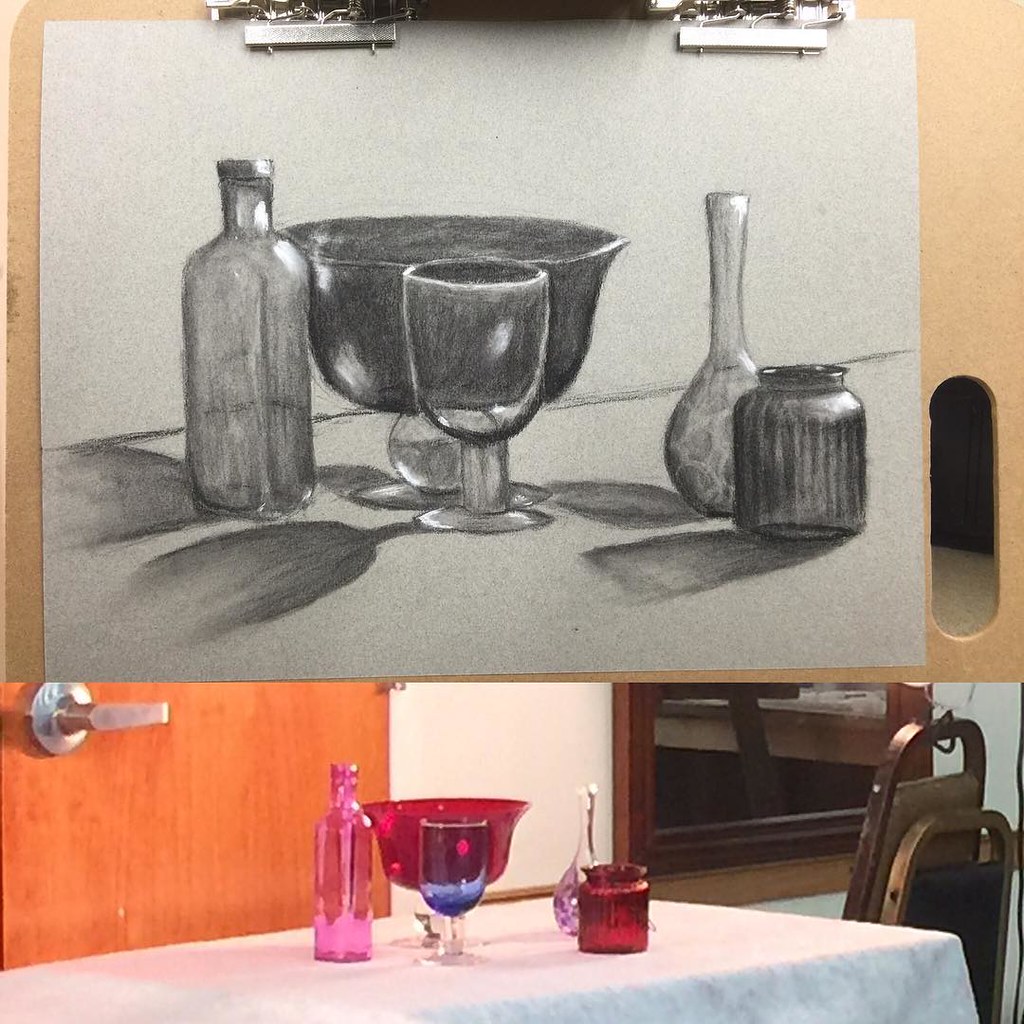The image is a collage consisting of two panels. The top panel features a pencil drawing clipped onto a wooden lap board with two silver clips at the top and an oval-shaped handle on the side. The drawing is of several objects, including a large bowl, a stemware glass, a long-necked bottle, a round-bellied bottle, and a small jar. The still-life is meticulously shaded in black and gray hues on white paper. 

The bottom panel is a photograph depicting the actual still-life arrangement inspired by the drawing. It shows the same objects—a red punch bowl, a blue stemware glass, a pink long-necked bottle, a purple round-bellied bottle, and a red small jar—arranged on a white tablecloth. This setup is placed in a room with a white wall, a brown wooden door with a stainless steel horizontal handle, and a mirror with a wooden frame. The table in the photograph is accompanied by at least two dark-colored, steel-frame chairs, further contextualizing the setting of the still-life display.